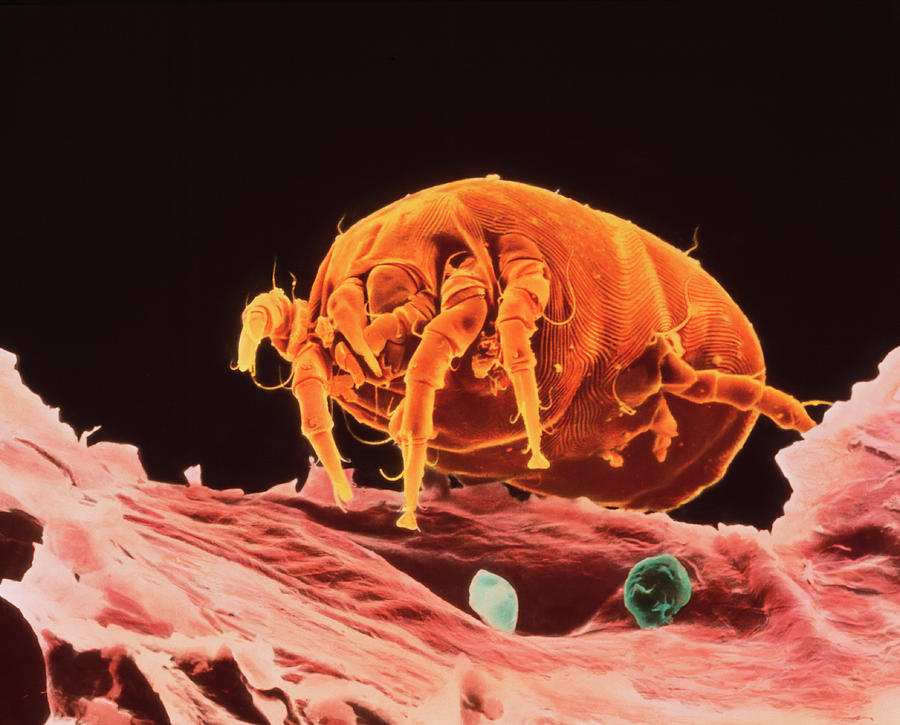Against a solid black background, this detailed, electron microscopic image reveals a bright orange, tick-like mite with a large, rounded body. The mite, featuring multiple legs and tiny wiry hairs, possesses two prominent front arms and longer back legs, along with a series of subtle ridges resembling a fingerprint on its back. Its face displays two to four small mandibles without any visible eyes. The mite is perched on a flaky, salmon and beige-colored surface, which resembles a skin cell flake. Surrounding the mite are small turquoise, teal, blue, and white granules scattered across the pinkish-brown tissue.